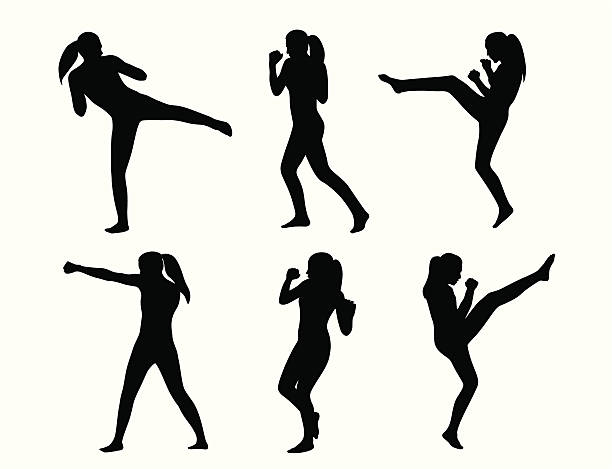The image is a compilation of six black silhouette figures of a woman with a long ponytail, depicted in various martial arts poses against a white background. Arranged in a 3x2 grid, the poses are as follows:

- **Top Row, Left**: The woman is seen from the back, executing a waist-height sidekick with her right leg, her arms positioned defensively in front of her.
- **Top Row, Center**: She is shown facing the left, with her feet planted firmly on the ground in a lunge position. Her right arm is extended in front of her face, forming a fist.
- **Top Row, Right**: The figure is captured mid-front kick with her right leg, her arms extended protectively in front of her chest.
- **Bottom Row, Left**: The woman stands with her legs apart, her left arm thrust forward in a fist, indicating a punching motion.
- **Bottom Row, Center**: She appears to be stepping back with her left leg, her right arm extended defensively in front of her face.
- **Bottom Row, Right**: The woman performs a high front kick with her right leg, her left arm raised defensively in front of her torso.

Each silhouette captures a dynamic moment, emphasizing fluid motion and martial arts technique.